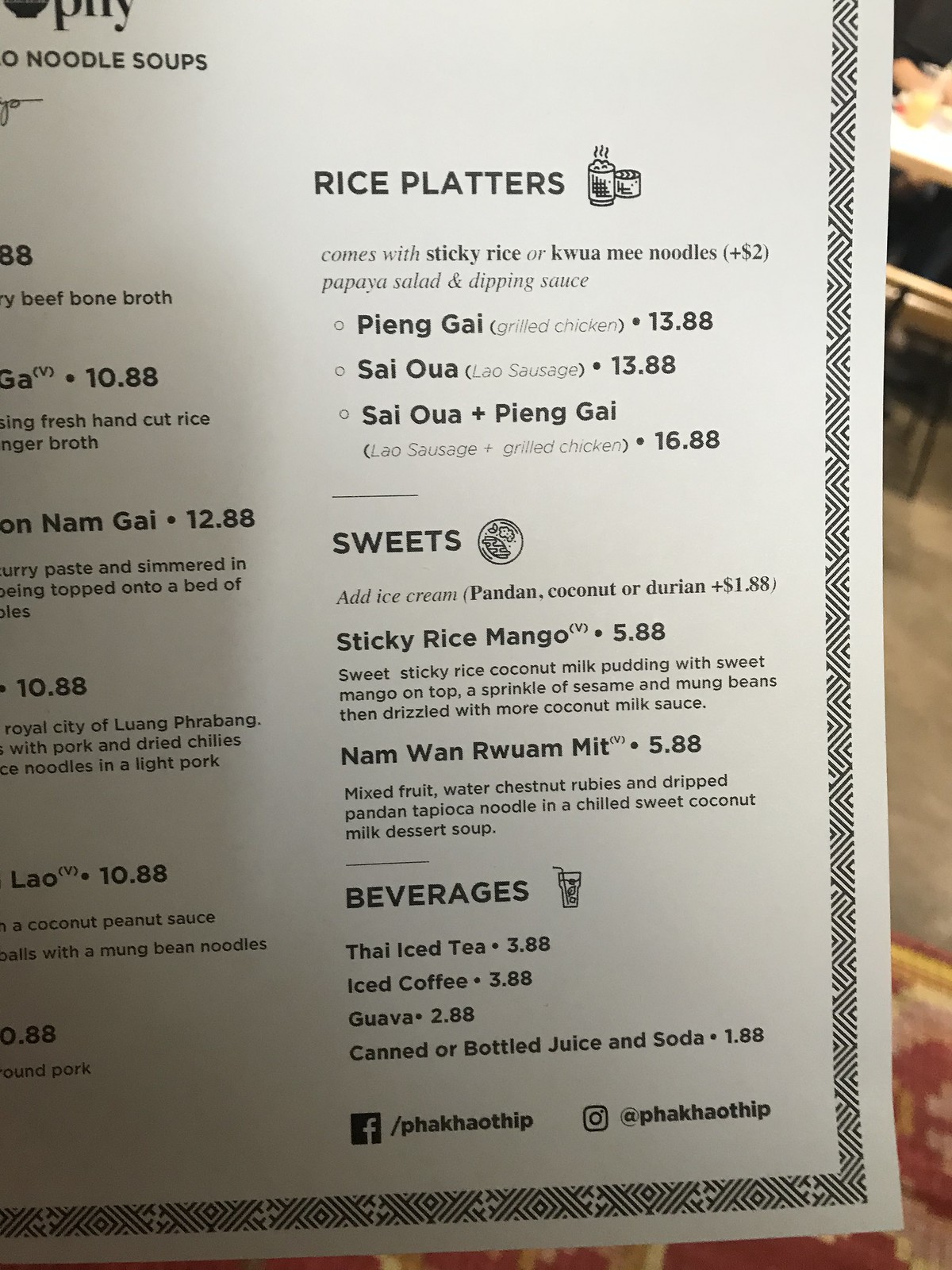The image depicts a menu from a Thai restaurant named Phakao Thiep. Although the entire menu isn't visible, the portions that are in view include sections dedicated to rice platters, sweets, and beverages. On the left side of the menu, one of the dishes, "Tom Nong Gai," is partially visible along with snippets of the entree section, suggesting a more comprehensive list exists beyond the cropped image. The rice platters offer options such as sticky rice or Kwame noodles, with dishes like Pheung Gai and Say Oi available. 

In the sweets section, delectable items like sticky rice with mango and Nam Wan Ruam Mit are listed. The beverage choices are equally diverse, featuring iced tea, iced coffee, guava juice, and various canned or bottled juices and sodas. The bottom of the menu prominently displays the restaurant’s social media tags for Facebook and Instagram, encouraging patrons to connect online.

The menu is held up inside the restaurant, evidenced by the faint background image of tables, adding a touch of authenticity to the scene. The visual presentation and item listings entice viewers with a glimpse into a delightful Thai culinary experience.